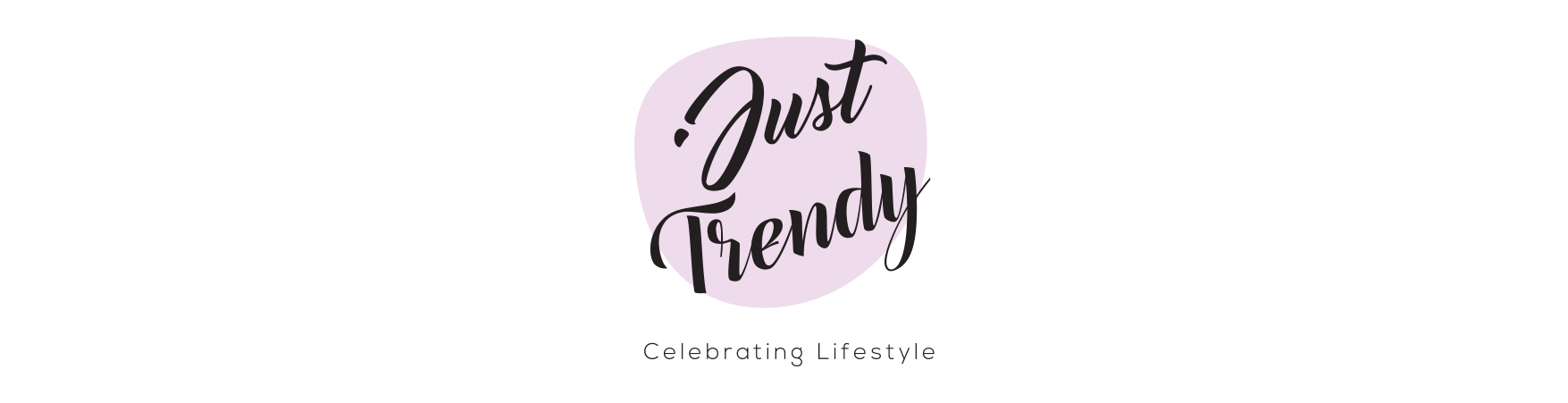The image showcases a company logo prominently centered against a pure white background. The logo features the words "Just Trendy" written in black cursive font, slanted slightly upwards, with "Just" positioned directly above "Trendy." These words are enclosed within an irregular, light purple circular shape, giving it a somewhat cartoony appearance. Below this circle, in small, printed black text, are the words "Celebrating Lifestyle," with only the first letters of each word capitalized. The logo's minimalist and stylish design makes it suitable for business cards or corporate websites.